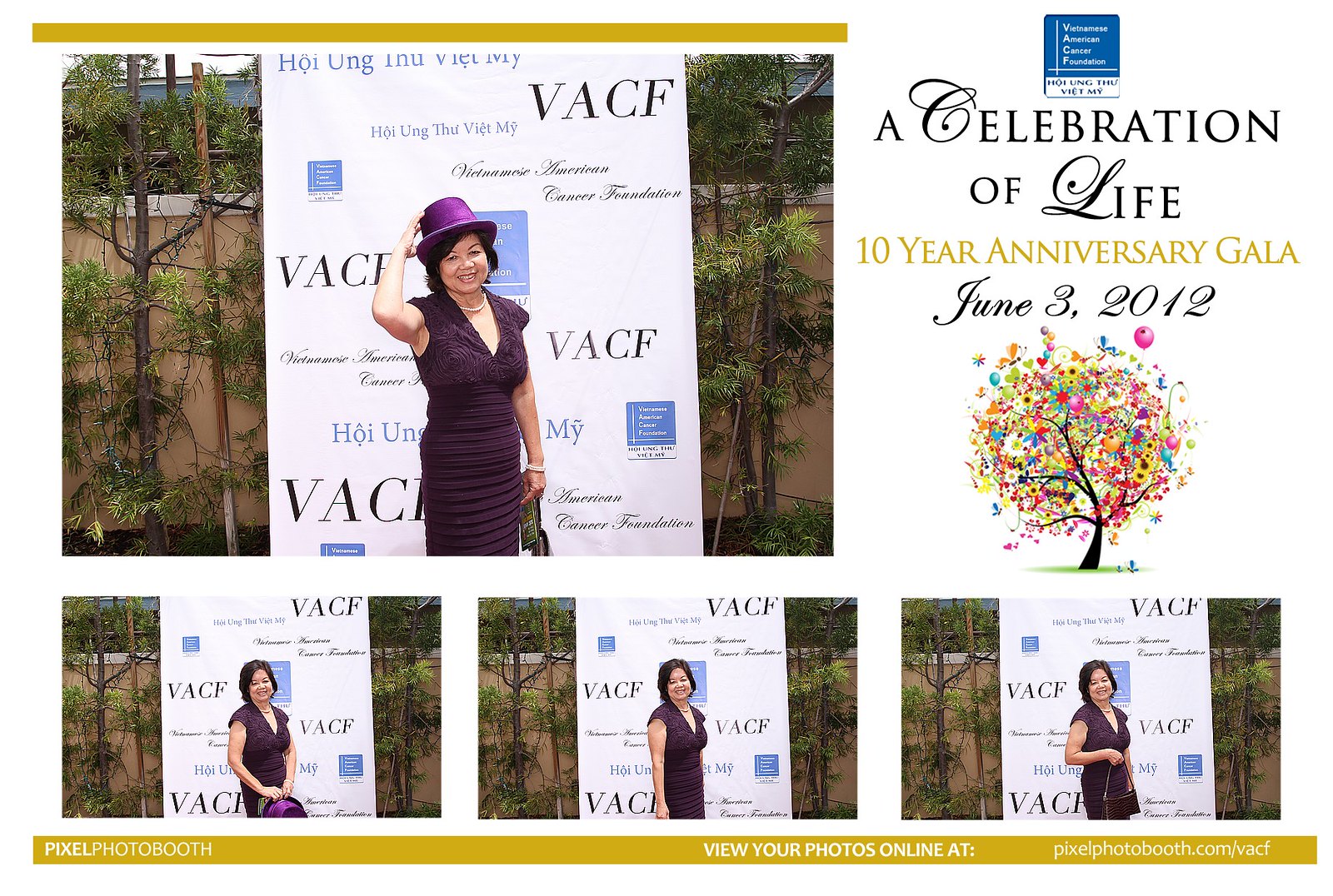This image is a photograph of an elegantly designed sign, created in honor of a woman, featuring a series of four photographs of the same Asian woman in a purple dress. The largest photograph, positioned at the top left, shows her wearing a purple hat and standing in front of a sign with Vietnamese text, "V-A-C-F H-O-I U-N-G T-H-U-L V-I-E-T M-Y," set against a backdrop of green trees and a brick wall. Directly below this, a smaller image captures her smiling while holding her hat. To the right of this, another photograph depicts her with arms at her sides, no longer holding the hat. The last image, in the far right corner, features her smiling and holding a pocketbook. The top right-hand corner of the sign includes a blue logo and text in blue and yellow that reads, "A Celebration of Life Ten Year Anniversary Gala June 3, 2012," adorned with a colorful tree design. The bottom of the sign includes a yellow border, with a watermark directing viewers to view their photos online at pixelphotobooth.com/V-A-C-F H-O-I U-N-G T-H-U-L V-I-E-T M-Y. The entire collection of images and text is arranged thoughtfully, creating a visually appealing and commemorative display.